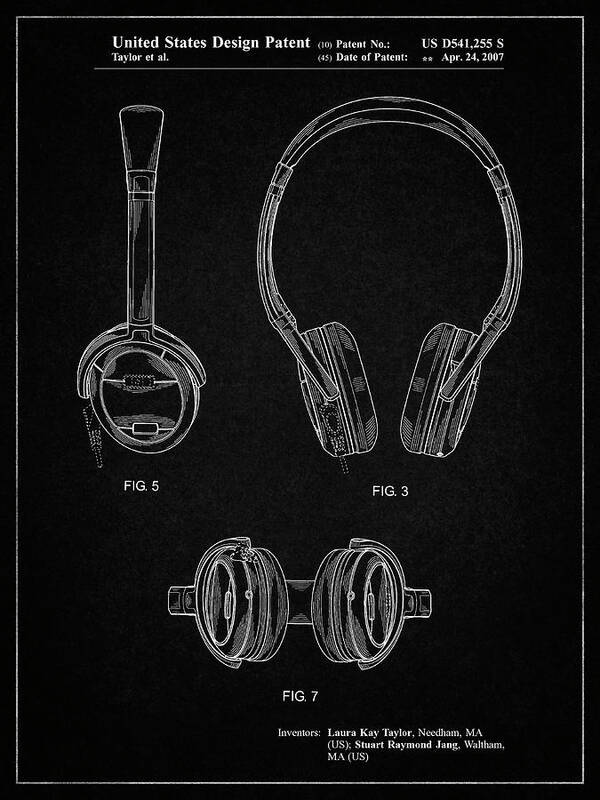This is a black and white illustration of a pair of over-the-head headphones, presented as a United States Design Patent. The background is black with all text and illustrations in white. The diagram features a white rectangular border with the heading "United States Design Patent" prominently displayed at the top along with the patent number USD541,255S and the date of patent, April 24, 2007. The central section of the diagram includes three labeled views of the headphones: "Figure 5" shows a side view, "Figure 3" presents a front view, and "Figure 7" depicts the bottom view of the headphones' ear pieces. At the very bottom, the inventors are listed: Laura K. Taylor from Needham, MA, and Stuart Raymond Jang from Waltham, MA. The overall presentation resembles white chalk drawings on a blackboard.